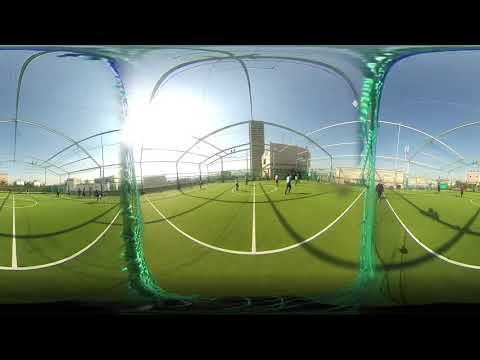The image depicts an outdoor soccer field with vibrant green turf marked by crisp white lines. Taken under bright sunlight, the clear blue sky forms a striking backdrop. Several people are seen running on the field, enclosed by fence poles casting dark gray shadows across the ground. The perspective is distinctly distorted, likely captured through a fisheye lens or perhaps even through netting, giving a rounded and magnified effect to the scene. Towards the left side of the image, the intense sunlight creates a washout effect, blurring some of the frame's details. Surrounding the field, there are numerous buildings in the background, including a notable square building and tall, rectangular tower. The image appears to be taken in a vibrant, bustling area with a mix of architectural elements and people engaged in an activity.